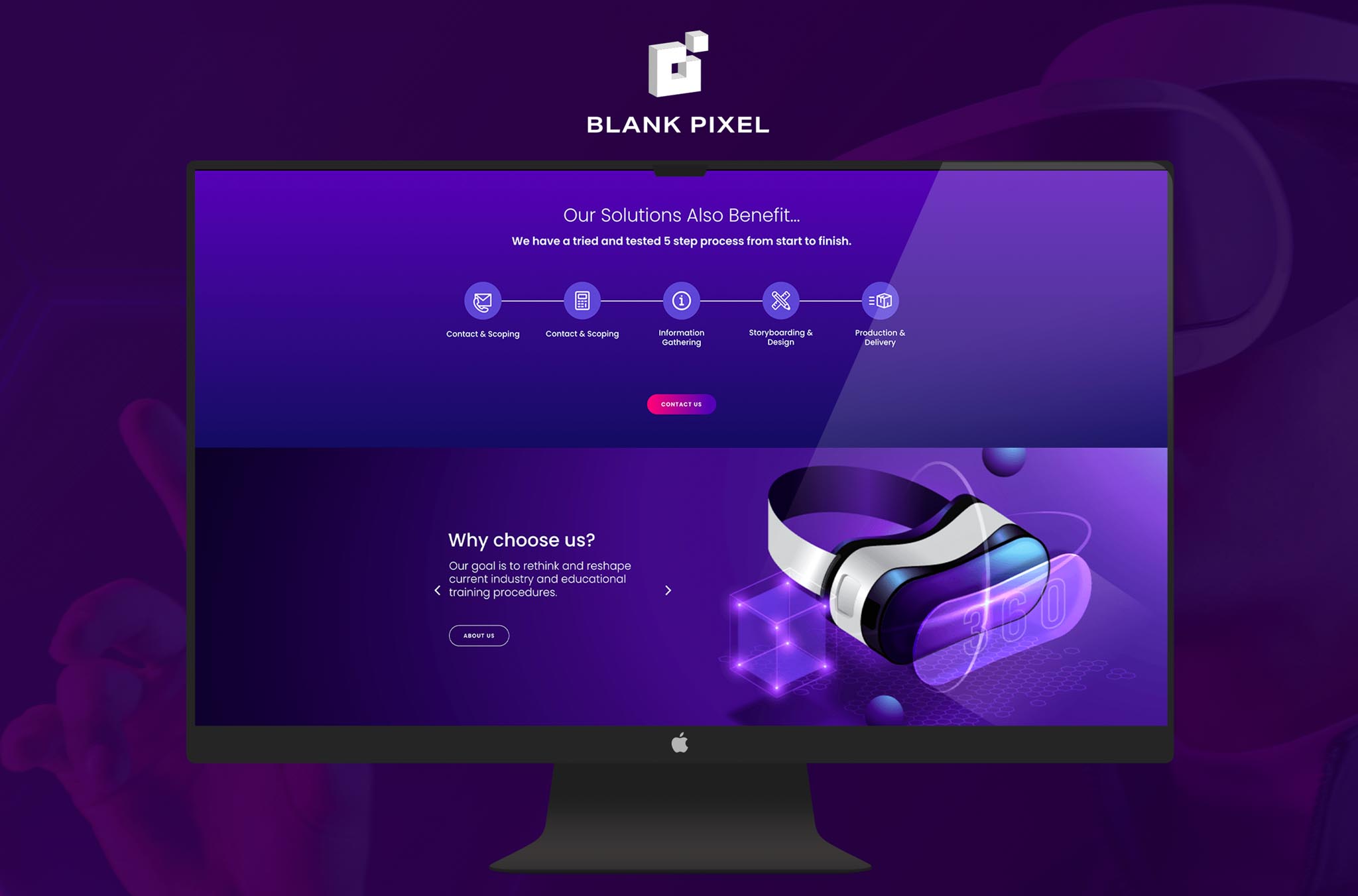The image features a predominantly purple background with various intricate elements. At the top, there's a square with a blank pixel inside. A central Apple monitor is prominently displayed, showing the iconic Apple symbol. The monitor's edges are black and it contains the text: "Our solutions also benefit. We have a tried and tested five-step process from start to finish." 

Below this text, a blue circle highlights the words "Contact and Scoping," and additional subheadings are listed: "First Gathering Process," "Storyboarding and Design," "Production," and "Delivery." 

An inscription reads: "Our goal is to rethink every aspect of engineer training procedures." Within this detailed layout, there's a graphic representation featuring a headset and a visor, labeled as "360 degrees," surrounded by spinning circles.

To the left side of the image, there's a queue with dots at its corners, giving off an island-like appearance, alongside various hexagons and circular shapes, creating an intricate and visually engaging scene.